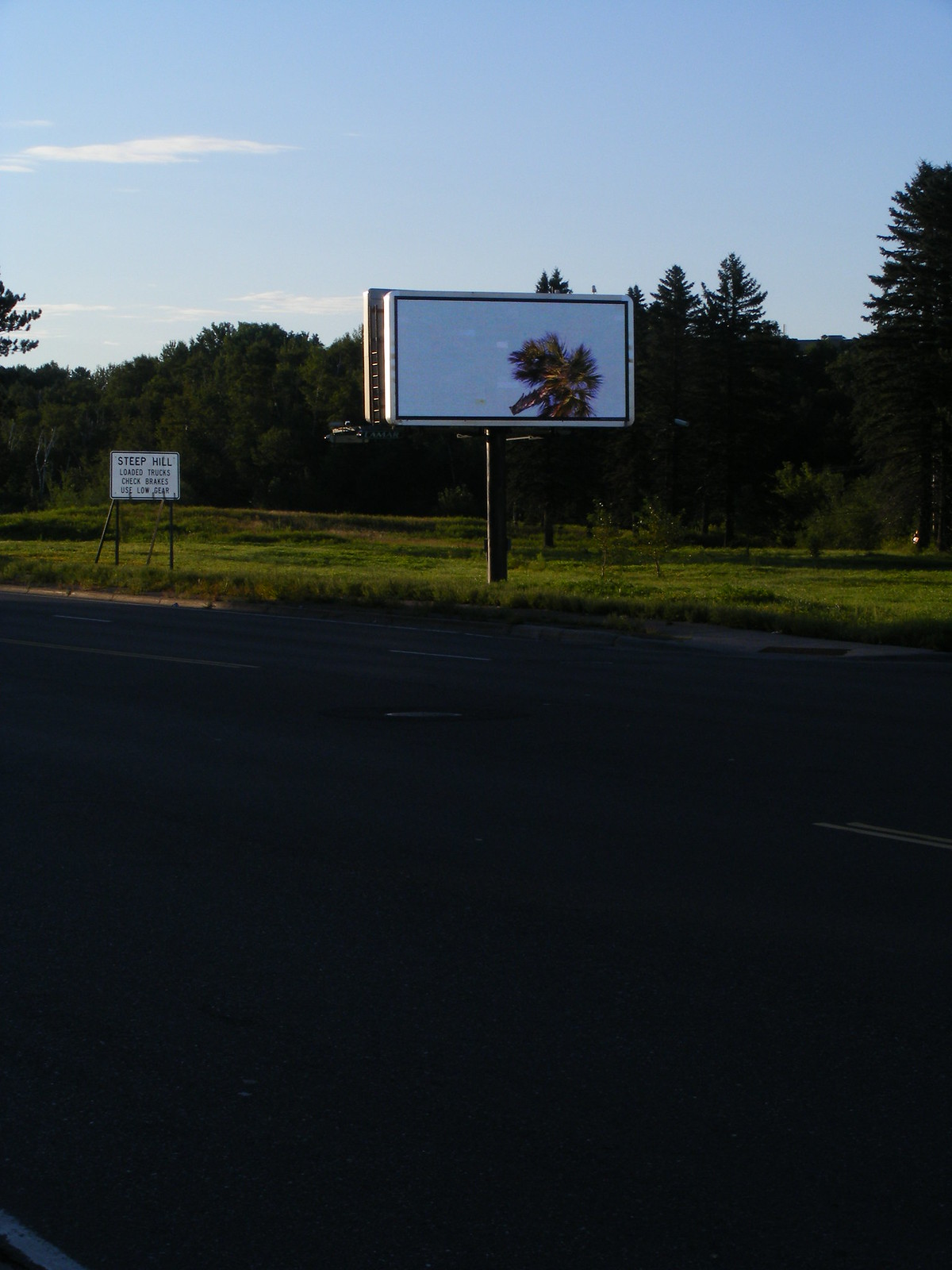The image is a vertical portrait orientation, approximately 50% taller than it is wide. Dominating the lower half of the image is a dark, almost black, angled road that extends to the bottom edge. The road, devoid of cars or lane markings, slopes gently from left to right at an approximate angle of 5 to 10 degrees.

Rising from the middle of the image is a billboard mounted on a single dark-colored post, estimated to be around 10 feet tall in real life. The billboard itself is a landscape rectangle with a white background, framed by a black border that does not extend to the very edges, leaving a thin white margin around the border.

In the lower right portion of the billboard, there is an indistinct shape that could be interpreted as either a squashed furry object, perhaps resembling an animal, or as a three-leaf clover or flower. This shape appears to be multicolored, with reddish and pinkish hues, but the overall darkness of the image makes it difficult to discern clearly. There are no words on the billboard.

Due to the angle, we can see part of the reverse side of the billboard as well. Behind the billboard is a dense thicket of dark green trees.

To the left side of the image, further down the road, there is a smaller rectangular sign with white background and black lettering. The top line reads "Steep Hill," followed by three lines of text too small to be legible.

The sky in the upper part of the background is light blue, adorned with a few scattered white clouds.